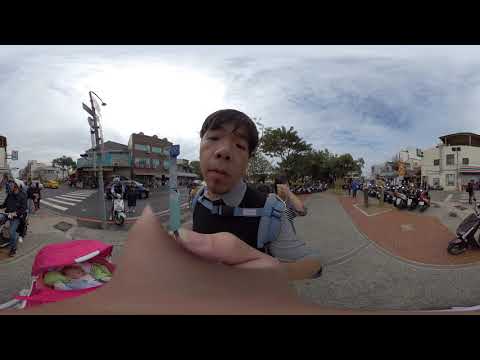This outdoor photograph, taken as a selfie, appears somewhat distorted and low quality, primarily affecting the foreground. The man, with short black hair, wearing a layered outfit of a button-down shirt, vest, and blue backpack, holds a selfie stick that magnifies his face and hand. Directly beside him, to the left, a baby sits in a pink stroller. The setting is a small city with low-rise buildings, ranging from second to third stories, with tan and terracotta-colored streets. To the right, a row of parked motorbikes adds to the urban feel. Several street signs and a crosswalk are visible, along with multiple pedestrians. The sky is mostly cloudy with some sunlight breaking through. The image dimensions are approximately five inches wide by four inches tall, colorfully capturing shades of black, blue, gray, white, pink, green, brown, and yellow.